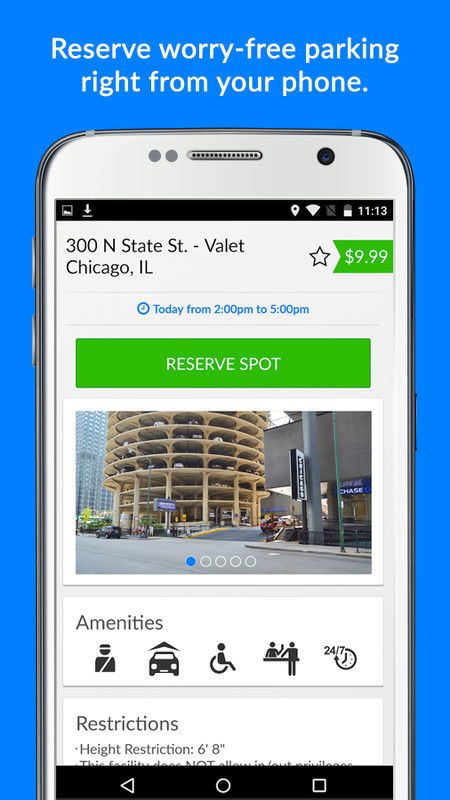This screenshot, likely from a smartphone, displays a blue background with white text that reads, "Reserved parking right from your phone." The image prominently features a smartphone, possibly an iPhone, displaying the time 11:13 without specifying AM or PM. The battery icon shows about 50% charge. At the top of the screen, it lists the address "300 North State Street, Valley, Chicago, Illinois," with a '999' icon to the right. Below this, it indicates a reservation for today from 2 PM to 5 PM, with a green "Reserve Spot" button. Additionally, there's an image of a parking garage, accompanied by the text "Amenities." Following this, there are icons representing a police officer, a car, wheelchair accessibility, and the numbers '24-7' and '9 o'clock.'